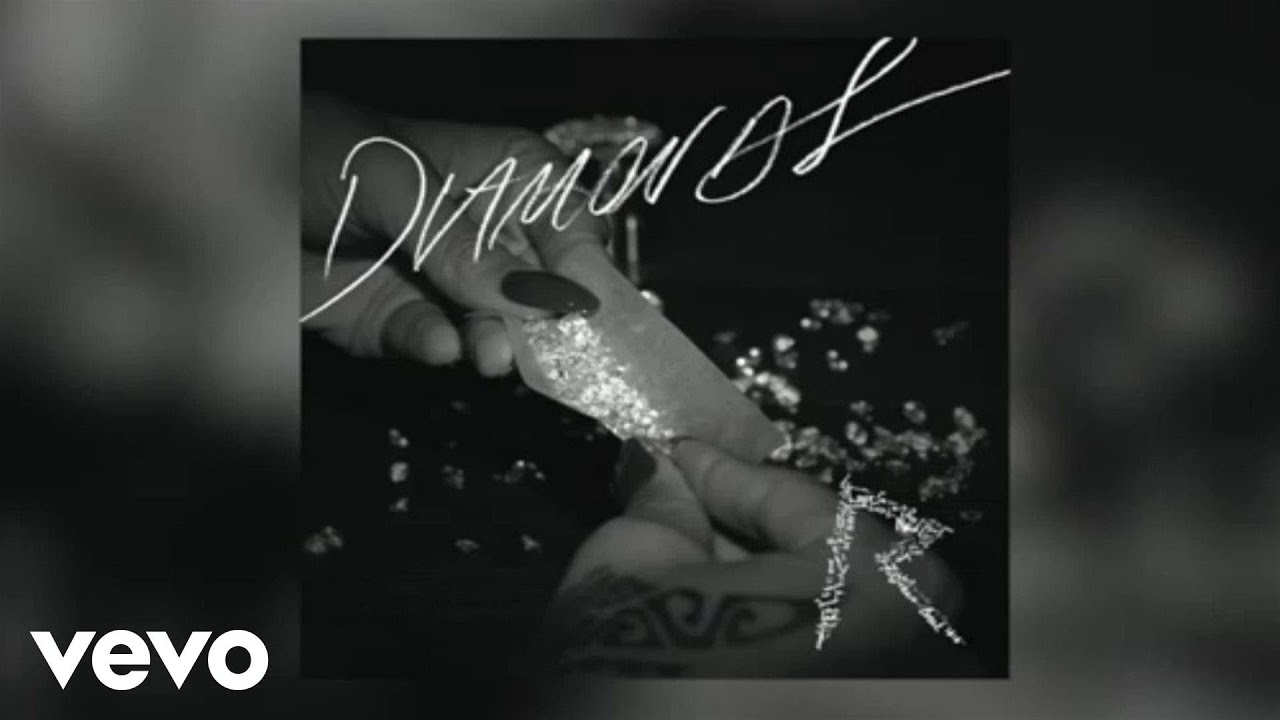The image appears to be a high-definition screenshot from a video on the music streaming website, VEVO, identified by the white "VEVO" text in the bottom left corner. Dominating the center is Rihanna's black and white album cover for "Diamonds." The cover features an elegant cursive "Diamonds" text and a stylized "R" in the bottom right corner, symbolizing Rihanna. The visual centerpiece shows two hands, likely Rihanna's—with one bearing a tattoo—rolling up diamonds in a small piece of paper, mimicking the preparation of a cigarette or blunt. Scattered diamonds lie beneath the hands on a table. The overall image is a blend of sharp focus on the album cover with a background of blurry grays and blacks, reinforcing the dreamy, high-production aesthetic typical of VEVO’s music video presentations.